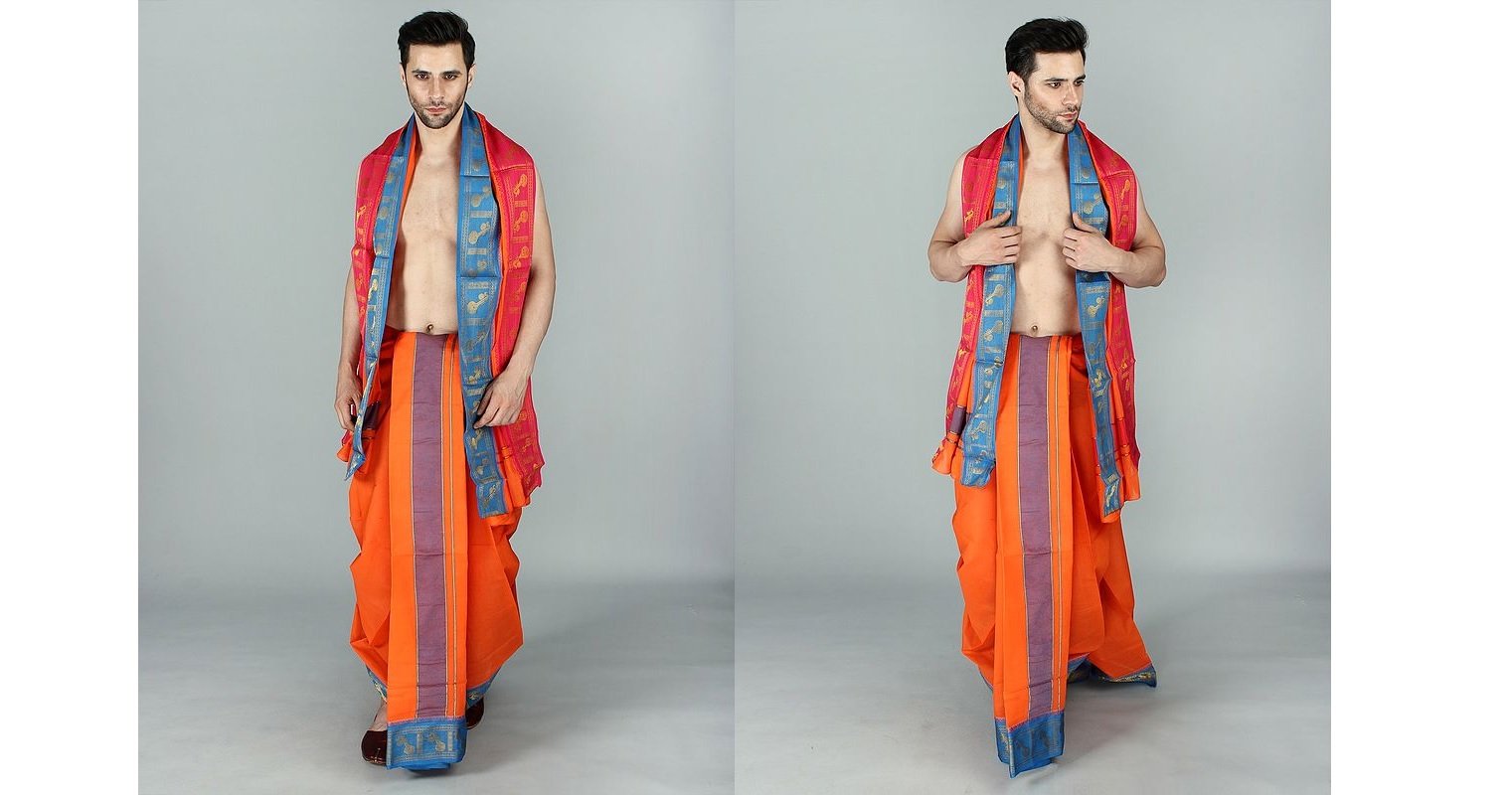The image features a young, white male appearing twice against a light gray background, with the picture split vertically to show two perspectives. In both sides of the image, the man is dressed in vibrant, traditional attire reminiscent of an Indian sari. He is shirtless, and his outfit comprises two main pieces: a vividly colored wrap that drapes over his shoulders, and an ornate skirt-like garment. The wrap is primarily red and blue with brown symbols, while the skirt, orange in color, features a distinctive purple stripe down the middle and blue at the bottom. He is also wearing black flat shoes. The left side of the image captures the man looking directly at the camera, showcasing his dark, neatly trimmed hair and a full but closely-cropped beard, giving him a professional and model-like appearance. In the right side, he poses with his head turned to the side, adding an element of dynamism to the composition. The overall impression is one of poised elegance and traditional yet striking fashion.